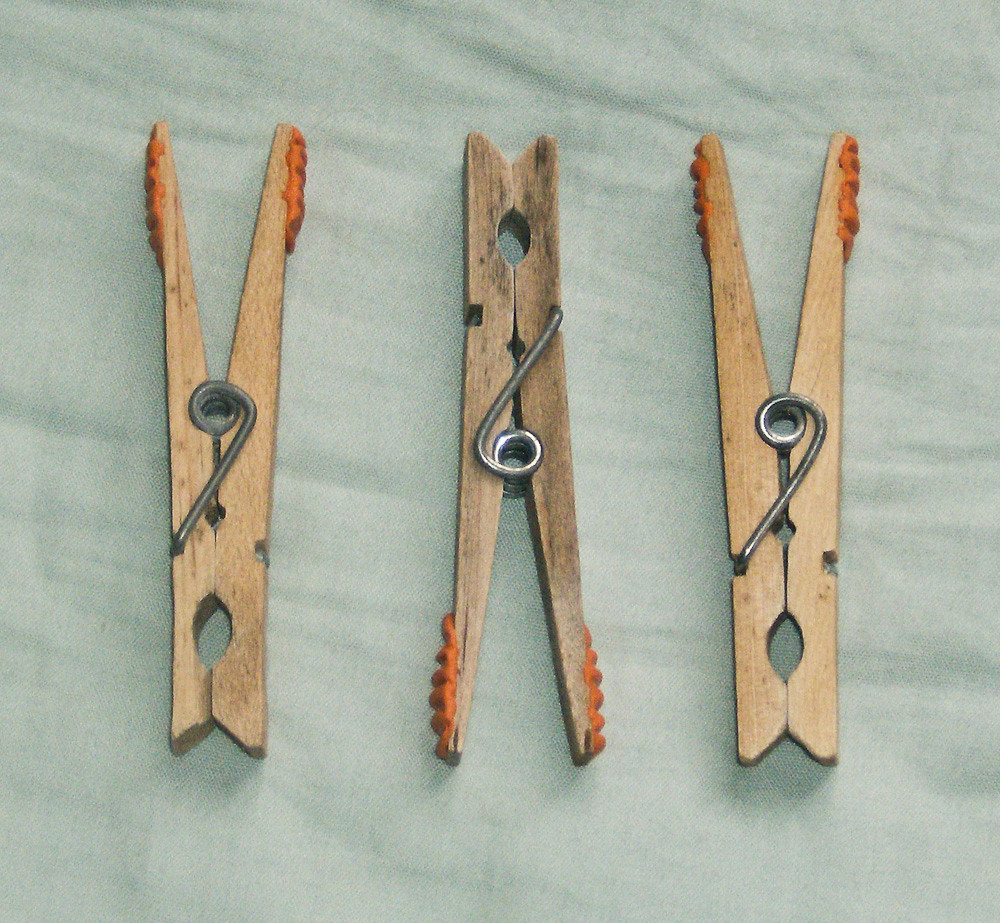This photograph captures an overhead view of three wooden clothespins resting on a light green, somewhat wrinkled cloth background. The clothespins are arranged in a parallel pattern, with the two outer ones facing downwards and the middle one facing upwards. Each clothespin is crafted from smooth wood, featuring a central metal spiral mechanism typical of traditional designs. The clothespins also have orange rubber-like grips at the handle ends. Notably, the middle clothespin displays a slightly darker wood tone compared to the lighter hues of the outer two. The detailed texture of the cloth and the even spacing of the clothespins create a balanced composition within the frame.